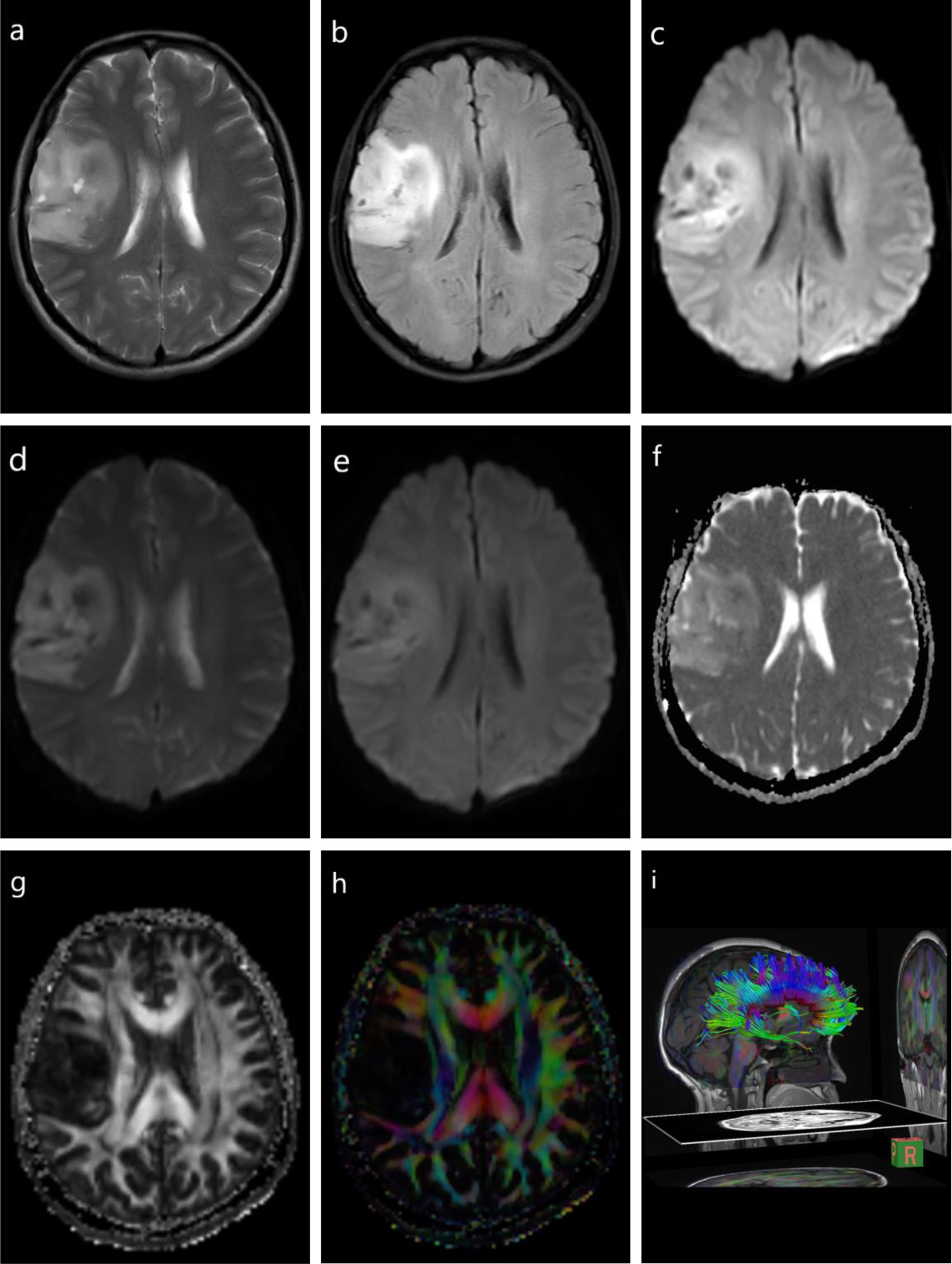This image comprises a series of nine different medical scans of the same human brain, arrayed in a 3x3 grid labeled A through I. The scans predominantly feature black-and-white imagery characteristic of MRI or CAT scans, with a noticeable tumorous growth present in the left-hand side of each scan. This abnormal area appears denser and more opaque compared to the surrounding brain tissue, which displays the typical gray-scale layers. The scans in the top rows (A, B, C) and middle rows (D, E, F) showcase varying degrees of gray and white contrasts, highlighting different aspects of the brain’s internal structure. Moving to the bottom row, the scans G, H, I transition into colored imagery. Specifically, in image H, the tumor remains a dark mass amidst bright colors like pink, green, blue, and orange denoting active brain regions. Image I presents a 3D rendering of the brain in profile view, integrating the same vibrant colors overlaid on the skull, emphasizing the detailed aspects of the tumor within the brain's overall anatomy.